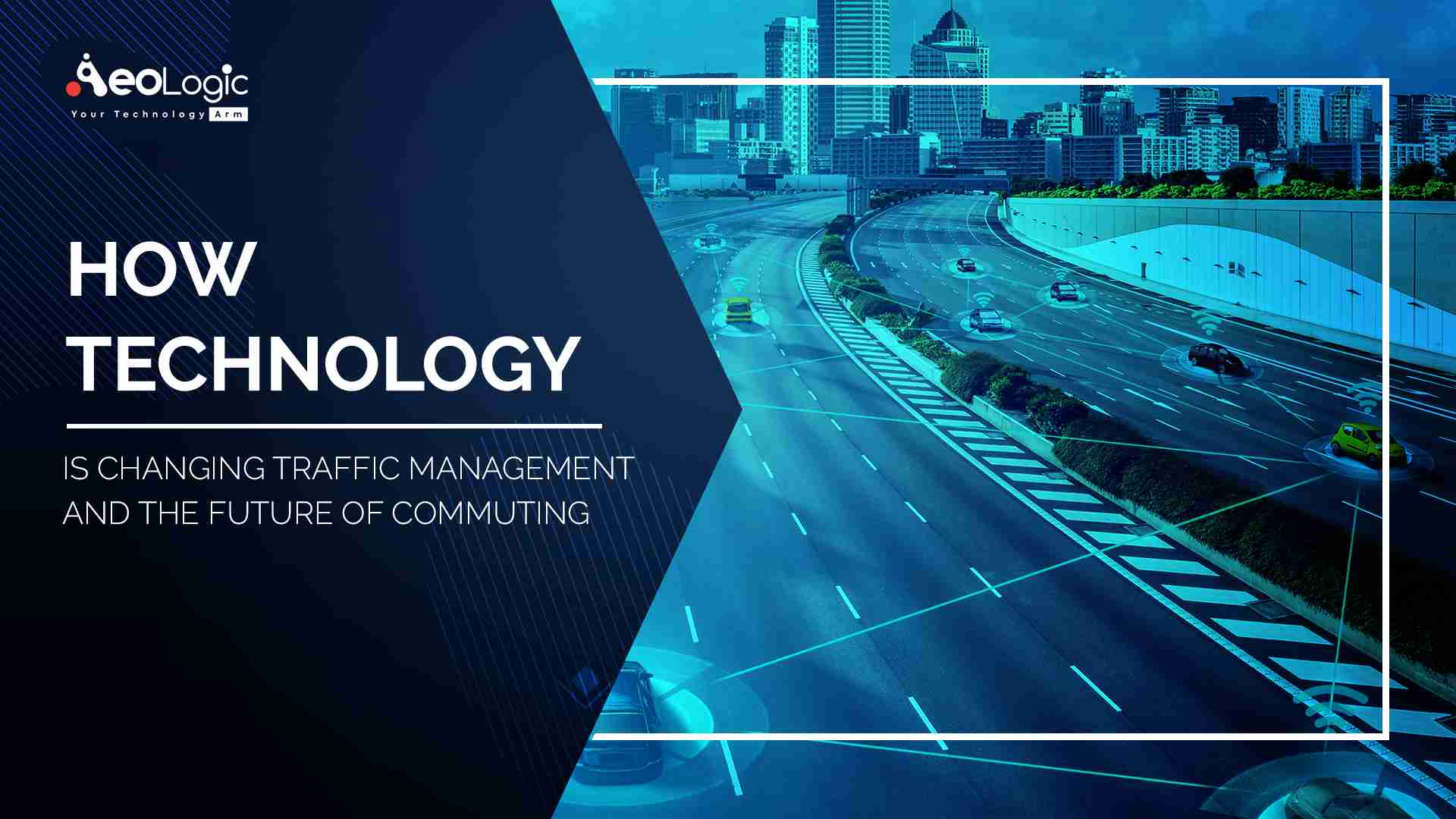The image depicts the beginning slide of a presentation by AeroLogic, highlighted in its logo on the left and right sides. The background is a cityscape with a highway and vehicles, filtered predominantly in shades of blue. The highway comprises six lanes on each side, divided by a barrier with trees, totalling ten lanes of traffic flowing in either direction. Several vehicles are shown, each with Wi-Fi signal symbols emanating from them, suggesting an emphasis on technological connectivity. Text on the left reads, "AeroLogic, your technology arm," and below, a headline states, "How Technology is Changing Traffic Management and the Future of Commuting," underlined for emphasis. The image employs blue shading with slight touches of green, particularly noticeable on the plants atop the barrier, contrasting against the otherwise muted city colors. This slide likely sets the stage for a discussion on advancements in commuting and traffic management technology.